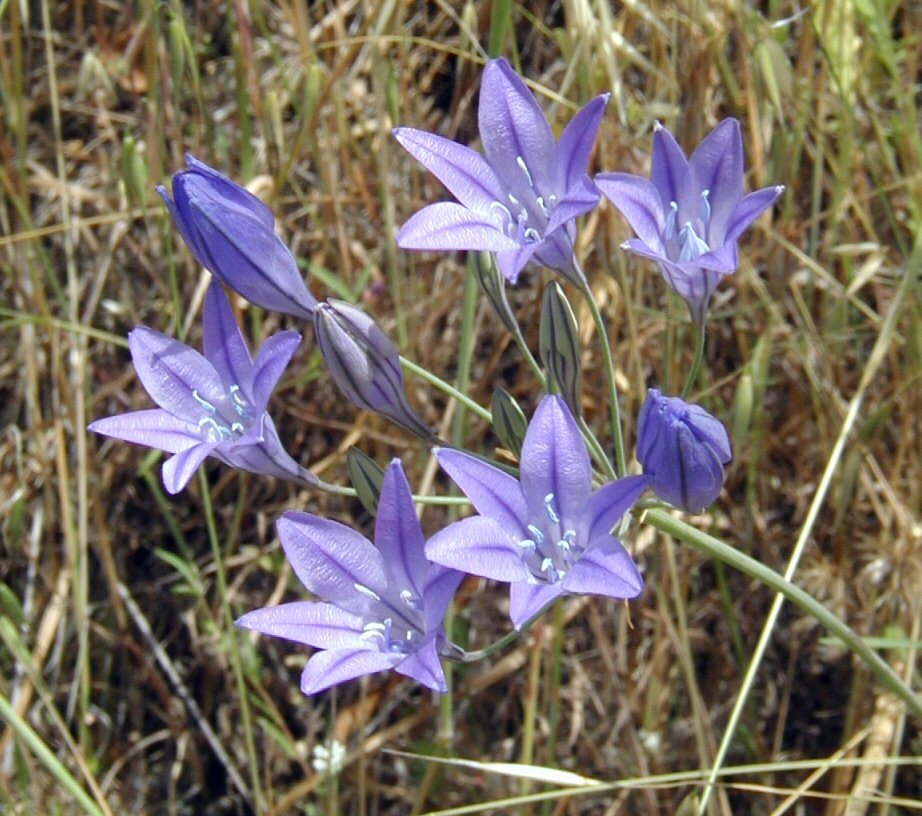In this detailed photograph, the main focus is a cluster of eye-catching purple lilies, each flower boasting six pointy yet slightly rounded petals. Along the length of each petal, you can see a darker purple streak. At the flowers' centers, numerous slender white stamens protrude, tipped with tiny, oval-shaped bulbs. The lilies are perched on light green stems which are accompanied by broad green leaves. The scene unfolds outdoors in what appears to be a swampy, marshy area. The backdrop is a tapestry of dry tan and golden-yellow reeds, interspersed with patches of green plant stems and brown soil, giving the impression of a wetland environment. Light seems to be filtering in from the upper left, casting a natural glow over the setting. The image is horizontally aligned, slightly wider than it is tall, capturing not just the vibrant lilies in sharp detail but also the blurred, crisscrossing grasses and reeds in the background, enhancing the depth and texture of the entire scene.